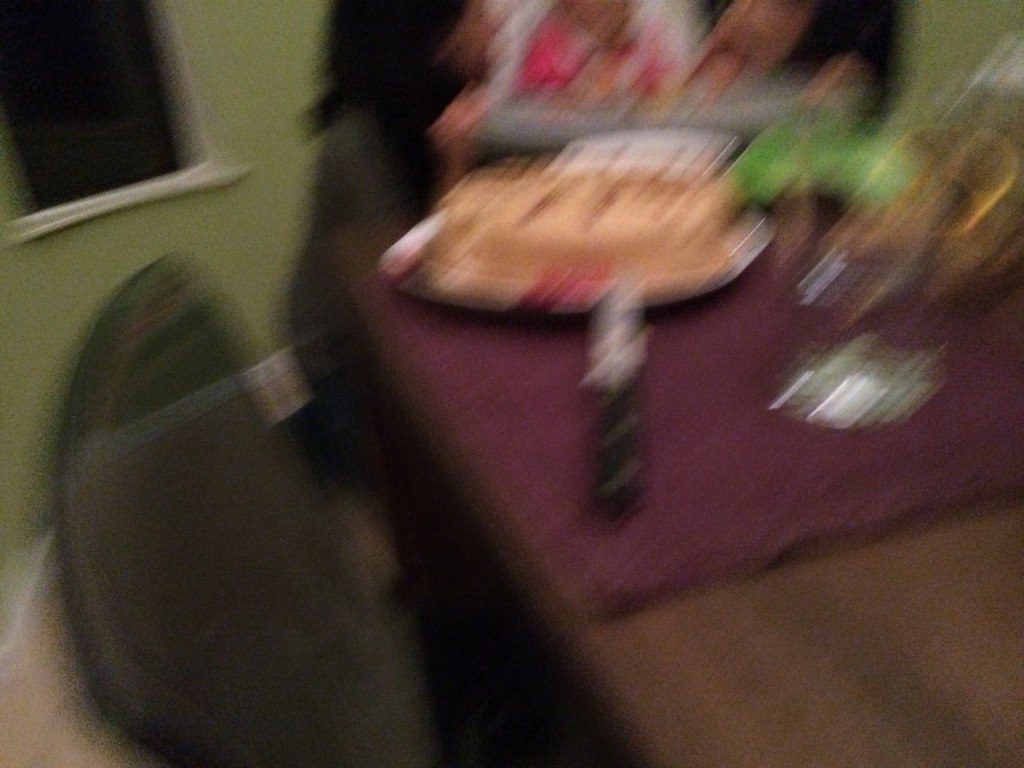The image appears to capture a highly blurry scene of what seems to be a birthday party. Central to the scene is a walnut dining table, partially covered with a purple tablecloth, upon which sits a birthday cake. The cake, possibly orange in color but indiscernible due to the blur, is placed on a white serving tray with a long white and black handle. A knife, ready for cutting, rests on the plate with the cake. The background features a green wall adorned with a window framed in white trim. To the left of the table is what looks like a wicker chair, discernible by the visibility of the white baseboard through its structure. 

The overall motion blur indicates the camera was rapidly moved from bottom to top at a 45-degree angle, rendering the photo largely out of focus. A pink dress, possibly worn by the guest of honor, can be seen behind the table. To the right, several color blurs—green, orange, and white—are present, and on the left, there is a large indistinguishable brown oval object in the corner. The room's walls are mostly an ivory white, with outside visibility limited due to darkness. Despite the blur and motion, the sense of a festive gathering centered around the cake is palpable.